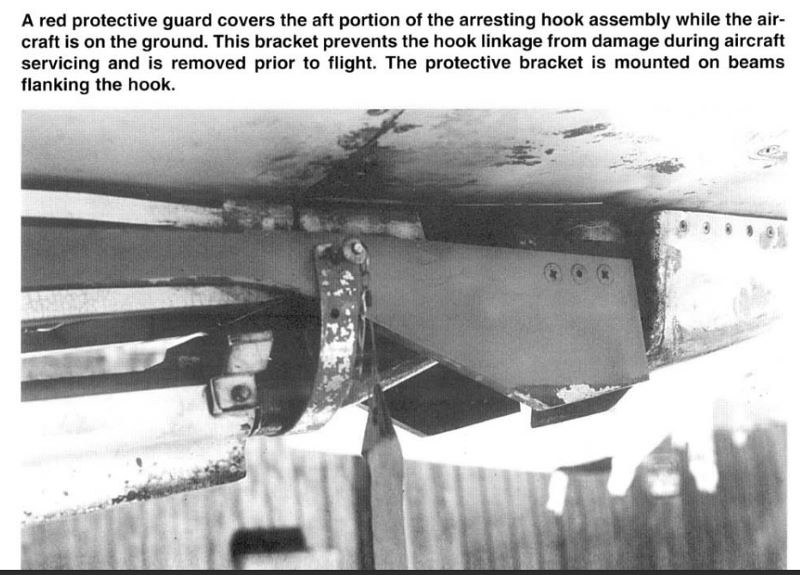The photograph appears to be a black-and-white image from an old book or magazine, possibly dating back to the 1970s. The top portion of the image features a paragraph in black font that reads: "A red protective guard covers the aft portion of the arresting hook assembly while the aircraft is on the ground. This bracket prevents the hook linkage from damage during aircraft servicing and is removed prior to flight. The protective bracket is mounted on beams flanking the hook." 

Below this text, the photo shows an up-close view of the underside of an aircraft, highlighting the mechanical components of the arresting hook assembly. Centered in the image is the metal hook mounted on beams, with pins holding various metal pieces in place. The metal components are a whitish color with parts appearing dark and rusty, indicating significant wear and tear, as well as grease and grime suggesting heavy use. The background is somewhat blurry, showing potential fencing or a metal wall, adding to the industrial feel of the setting.